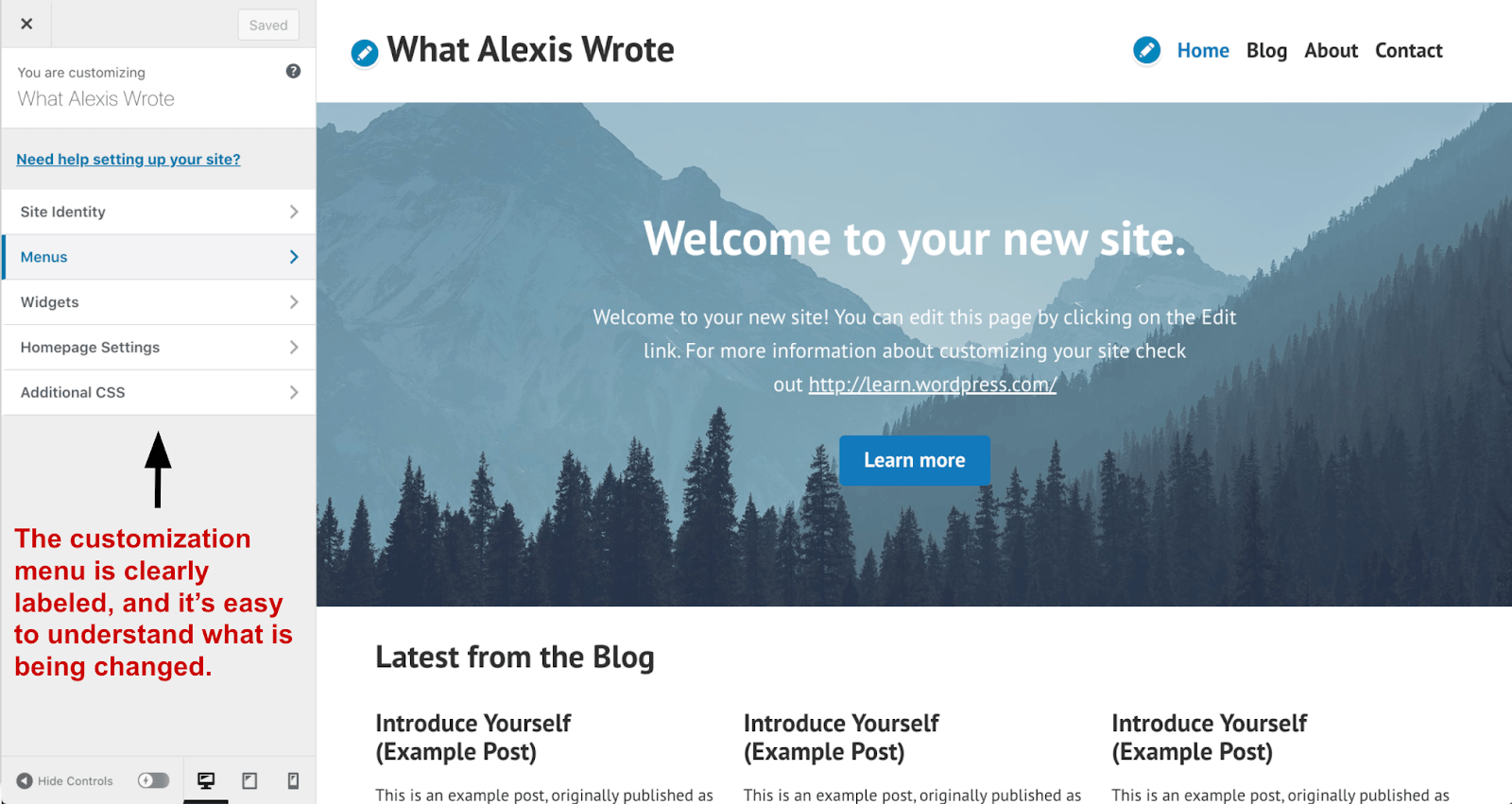**Screenshot of Blog Customization Interface**

The image showcases a detailed screenshot of a blog customization interface. On the left-hand side, a vertical bar titled "You are customizing What Alexis Wrote" prompts the user with "Need help setting up your site?" Several customization options are listed below, including Site Identity, Menus, Widgets, Homepage Settings, and Additional CSS. Encased in a gray box at the bottom, red text reads, "This customization menu is clearly labeled and it's easy to understand what is being changed." A black arrow points from this text to the individual customization options. 

On the right-hand side of the screen, the blog's preview is visible. The title "What Alexis Wrote" is prominently displayed at the top in black letters. The upper right section includes a navigation menu with options: Home (highlighted in blue as it is selected), Blog, About, and Contact (all in black). Below the navigation, there is a horizontal background image featuring a misty mountain landscape with green trees scattered throughout, overlaid with white text that reads, "Welcome to your new site." Below this message is an instruction to edit the page via an edit link, alongside a URL for more information (http://learn.wordpress.com). A blue button labeled "Learn More" is positioned beneath the welcome text.

At the very bottom of the preview, there's a section titled "Latest from the Blog," featuring repeated placeholder text for a post: "Introduce yourself, example post."